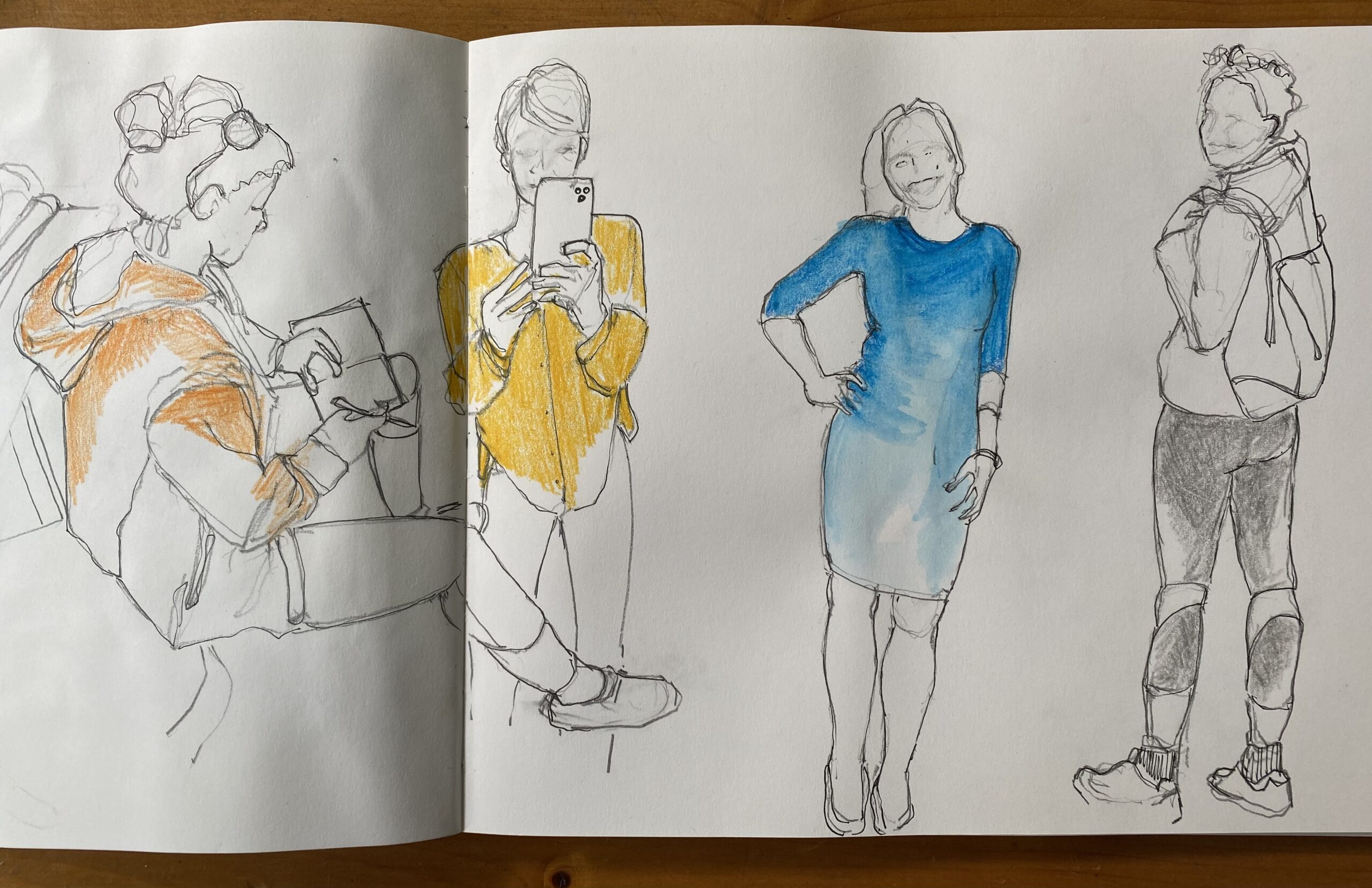This image captures the inside of a landscape-formatted drawing book, showcasing sketches of four women with various details and light coloring. The book is opened with a visible crease leaning towards the left side, making the right page more prominent. On the left page, a woman is seated, likely on a couch or bed, wearing an orange jacket with the top part colored. She has her hair pulled back and sunglasses on her head, focusing on an open book in front of her as if writing or sketching. Her foot extends slightly into the right page.

The remaining three women are primarily on the right page. The first, whose shoulder overlaps the crease, has short hair and is dressed in a yellow blouse. She appears to be using her phone, either taking a selfie or reading something. Next is a woman in a blue dress with high heels and a bracelet on her left arm, looking forward with a slight smile. The final woman, situated on the far right, stands with her back partially turned towards the viewer, her head tilted back showing a smile, and she is wearing a backpack. The shading and penciling techniques highlight initial stages of color, giving life to the outfits worn by each woman: the blue dress, the yellow blouse, and the orange jacket.